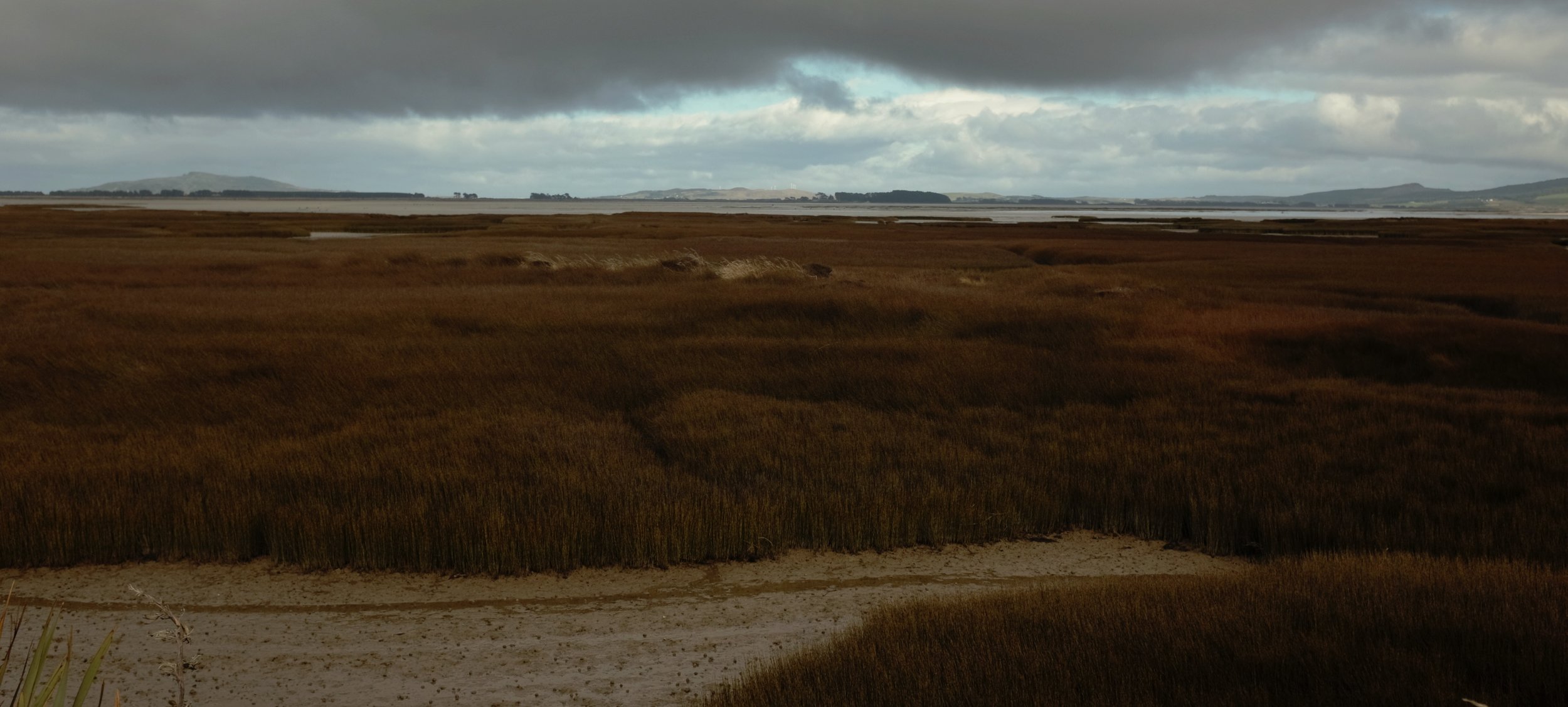In this scenic image, a vast, flat landscape stretches out under a moody sky. The foreground features a sandy, eggshell-beige area dotted with dark brown specks, where no vegetation grows. Surrounding this sandy patch and extending into the distance is a scrubland filled with tall, fluffy, dark brown grass. There is a narrow path or road visible near the bottom left of the image. The land is devoid of trees and buildings, maintaining its barren and almost desert-like appearance. In the far background, low mountains rise sparsely against the horizon. The sky overhead is layered with shades of blue and filled with ominous, low-hanging, dark gray clouds, suggesting imminent rain.